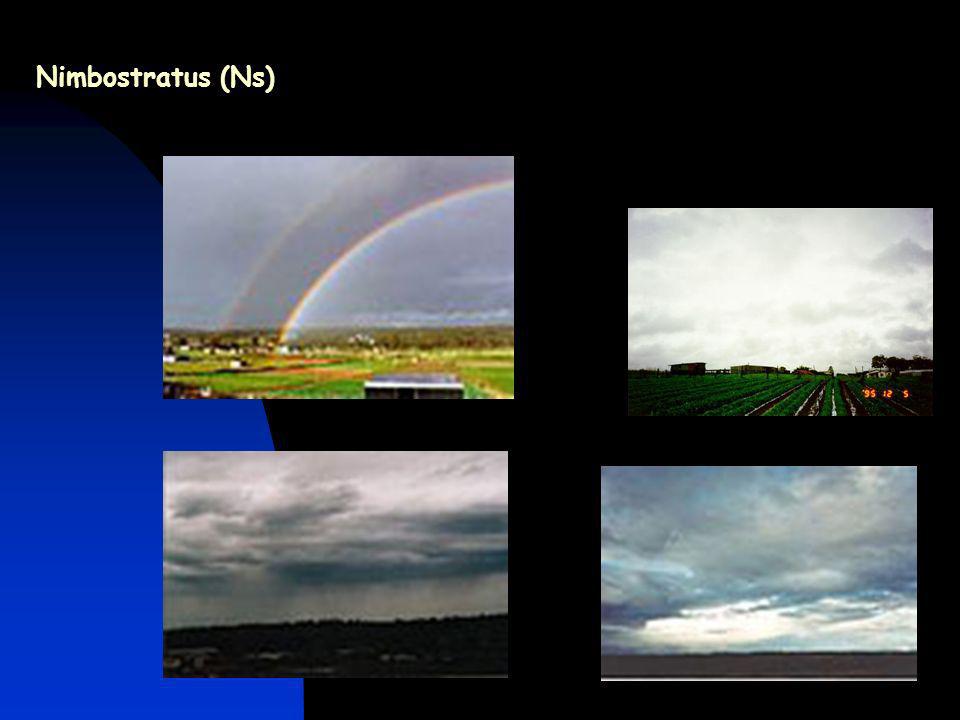This poster, titled "Nimbostratus" in bold yellow text in the top left corner, features a collage of four cloud-themed photographs set against a striking background. The background transitions from a gradient blue circular shape on the left to a stark black on the right, creating the effect of a planetary view. The image in the top left of the collage captures a vibrant rainbow over a farm, set beneath heavy cloud cover. To its right, the top right photograph also depicts a farmland scene blanketed by thick clouds. The bottom left shows an expanse dominated by clouds with a sharp black horizon beneath, giving a sense of endless sky. The bottom right mirrors this with another cloudy sky above a subtle horizon. The text "embossed dress ns" is subtly placed in white in the upper left section of the background, enhancing the ethereal and expansive feel of the poster.